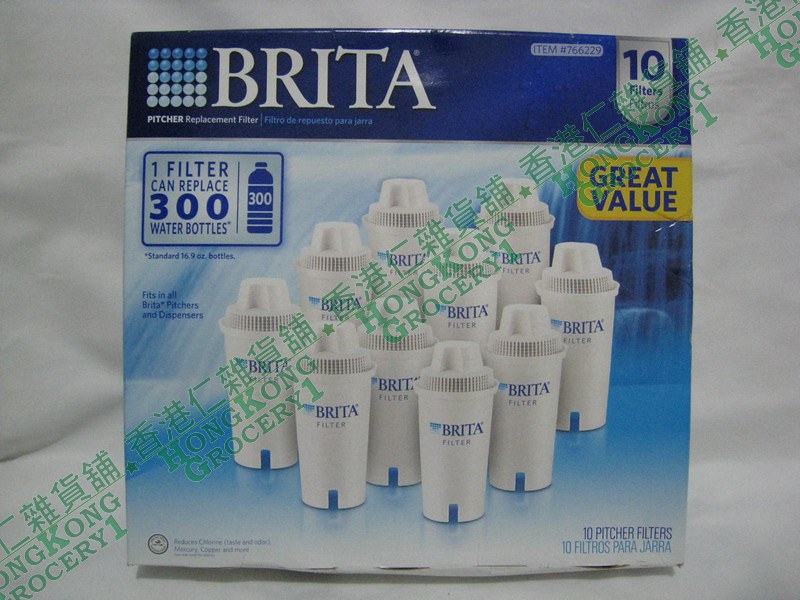This image features a horizontally oriented, color photograph of a Brita replacement filter box. The backdrop is a soft, white drapey cloth, reminiscent of a studio setup, providing a clean and professional background. The box itself has a bottom three-quarters in light blue and a top quarter in dark blue. Prominently displayed in large white font at the top left is "Brita," followed by a smaller description "picture replacement filter." Below that, a message in white lettering states that "one filter can replace 300 water bottles," with a small blue water bottle graphic indicating "300."

On the right side, a small white tab with blue text highlights "10 filters," and in the top right corner, a yellow sign with blue text states "great value." The front image on the box shows ten white Brita filters aligned in a pyramid formation, each labeled with the blue "Brita" text. Additionally, there is a watermark diagonally across the image in green Chinese characters accompanied by the text "Hong Kong grocery," indicating it may be a product image from a website. The item number "766229" is also mentioned on the box.